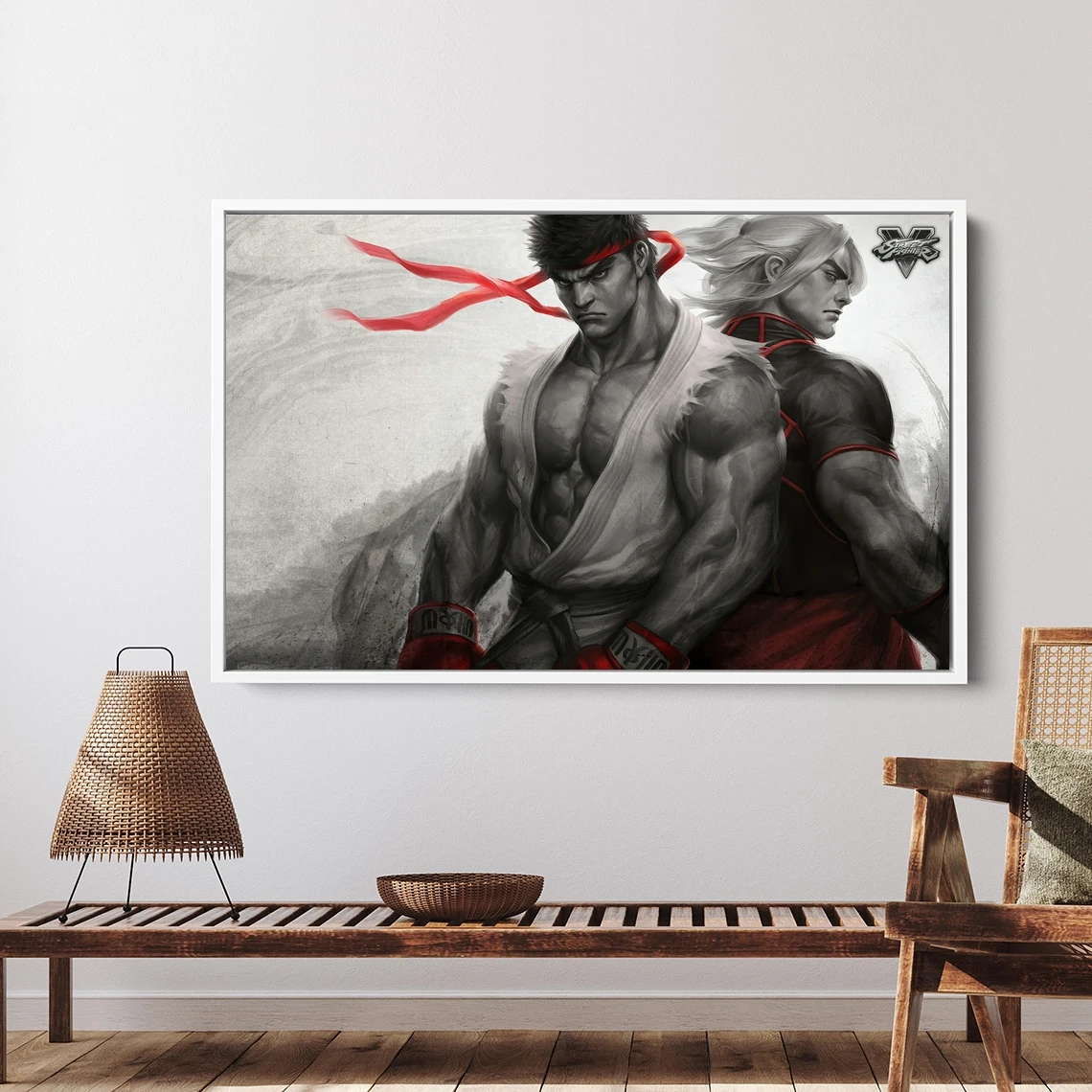The image is a detailed photograph taken indoors, showcasing a corner of a well-decorated room. The setting features a light gray wall with a low-level bench, fashioned from slatted wood, positioned centrally against it. The bench, adorned with a wicker bowl and a three-pronged wicker lamp on the left side, might also be interpreted as a table. To the right of the bench is a wooden chair with a gray throw pillow and a wicker backrest.

Dominating the focus of the image is an expansive, square-shaped painting with a white frame, occupying almost half of the wall space. The artwork depicts two muscular characters from the video game Street Fighter, rendered primarily in shades of gray. The character on the left, with brown hair and a red ribbon whipping in the wind around his head, faces towards the right, sporting a tattered vest and exhibiting a robust chest. The character on the right, clad in a black shirt and red bottoms, has white hair. The backdrop of the painting includes a gray sky and mountainous terrain, adding to the dramatic effect.

The floor beneath the setup is made of vertical brown wood slats, and light filters into the space from the left side, likely through a window not visible in the image. This composition creates a vivid, detailed scene that draws attention to both the furnishings and the striking central artwork.